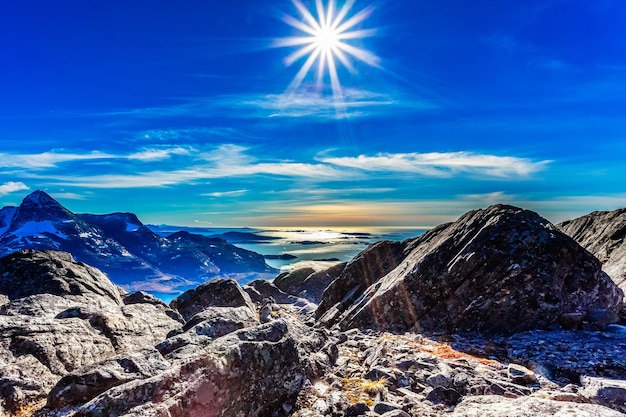This image captures a breathtaking, high-elevation, rocky mountaintop landscape with a mesmerizing play of light and shadow. In the foreground, the terrain is covered with a mix of black, gray, and brown boulders, speckled with bits of white. To the left, a tall mountain appears to be partially snow-covered, while on the right, a flat, snow-covered expanse stretches into the horizon, giving an almost barren appearance. The sky above is a vivid medium blue, adorned with wisps of white clouds. Dominating the upper center of the image is a bright, white sun, with its radiant beams extending outward, creating a striking visual effect on the landscape below. These beams selectively illuminate parts of the hills and rocks, casting dynamic shadows and enhancing the contrast between the sunlit and shaded areas. The whole scene evokes a sense of serene isolation, where natural elements interplay harmoniously under the clear, vibrant sky.